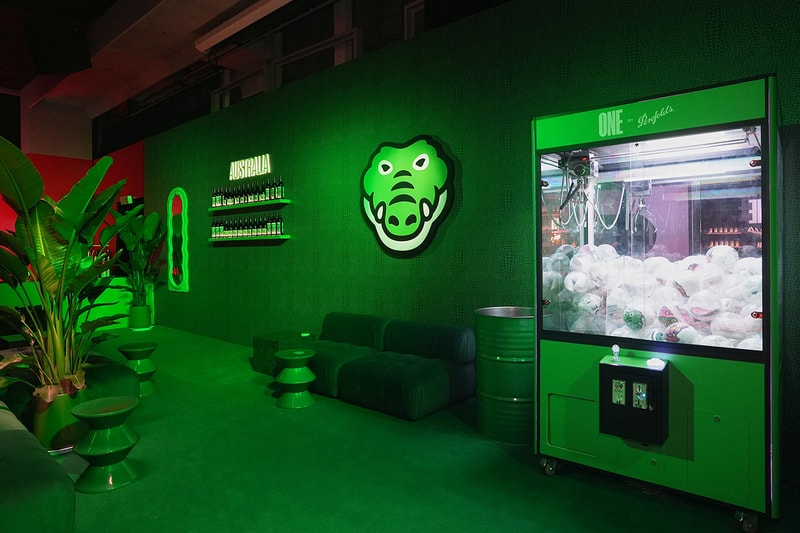The photograph captures an interior space that appears to be a game room, predominantly rendered in various shades of green. The entire right side of the image is dominated by a green claw machine, lit brightly on the inside, containing numerous orb-shaped items or balls featuring characters. Situated next to this machine is a green metal trash can with a silver interior, followed by a low-back green couch. Above the couch, a lit neon sign depicting a cartoonish alligator head adds a playful touch. Adjacent to the alligator sign are two green shelves mounted on the wall, holding small bottles, with the word "Australia" illuminated above them in white lettering. Below and to the left of the shelves is a narrow green mirror. The room also features movable green wooden side tables, which look like plant stands, and a large potted green plant. Although the entire room is immersed in green hues, the far-left wall introduces a contrasting red color. The ceiling reveals visible concrete pillars and overhead rafters. This eclectic mix suggests that the space may be a student activity room on a college campus.